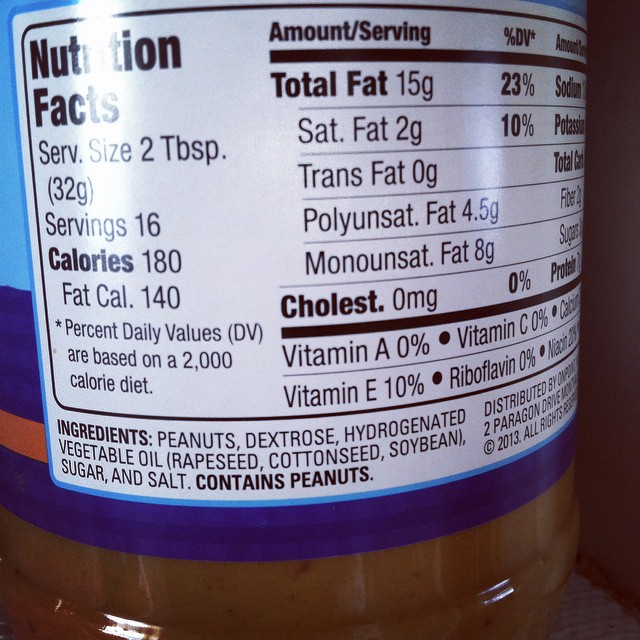A small bottle of peanut butter with a distinctive label is visible in the image, prominently displaying its nutritional information. The bottle contains 16 calories per serving, with a serving size of two tablespoons. However, it is notably high in calories, boasting 180 calories per two-tablespoon serving. The nutritional details indicate it provides 23% of the daily recommended value for total fat and 10% for saturated fat. The ingredient list highlights the presence of peanuts, dextrose (sugar), hydrogenated vegetable oil (made from rapeseed, cottonseed, and soybeans), sugar, and salt. The label is designed with a blue background and an orange stripe at the bottom. Visible through a window or door to the left, natural light illuminates the bottle, enhancing the clarity of the white and black nutritional information and ingredients. The product inside appears darker than typical peanut butter, hinting at its rich, high-fat content.